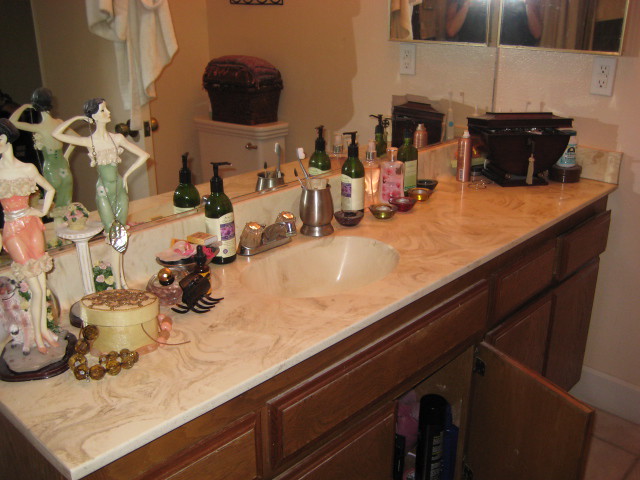This image captures a detailed view of a bathroom counter taken from an angled perspective, extending from the bottom left to the bottom right of the frame. The counter is crafted from white marble with distinct swirling patterns. It's a substantial, elongated counter featuring a single sink positioned centrally, adorned with vintage-style hot and cold knobs.

The cabinetry below the counter is a rich medium oak, offering a warm contrast to the marble surface. The arrangement consists of four lower cabinets topped by four upper drawers, providing ample storage.

The countertop is cluttered with various items. There are bottles of lotion and hand soap, as well as a hair clip scattered on the surface. Adding a touch of decorative elegance, the counter is adorned with slender porcelain figurines of women. One figurine, dressed in green, poses with one hand behind her head and the other on her hip. Another figurine, clad in orange, complements the scene.

On the wall to the right, mounted above the counter, is a medicine cabinet. A mirror behind the sink reveals a partial reflection of the person taking the picture, identifiable by a black shirt and a white arm. Notably, the upper portion of the reflection is cropped out. Completing the scene, a toilet is visible in the background, situated adjacent to the sink.